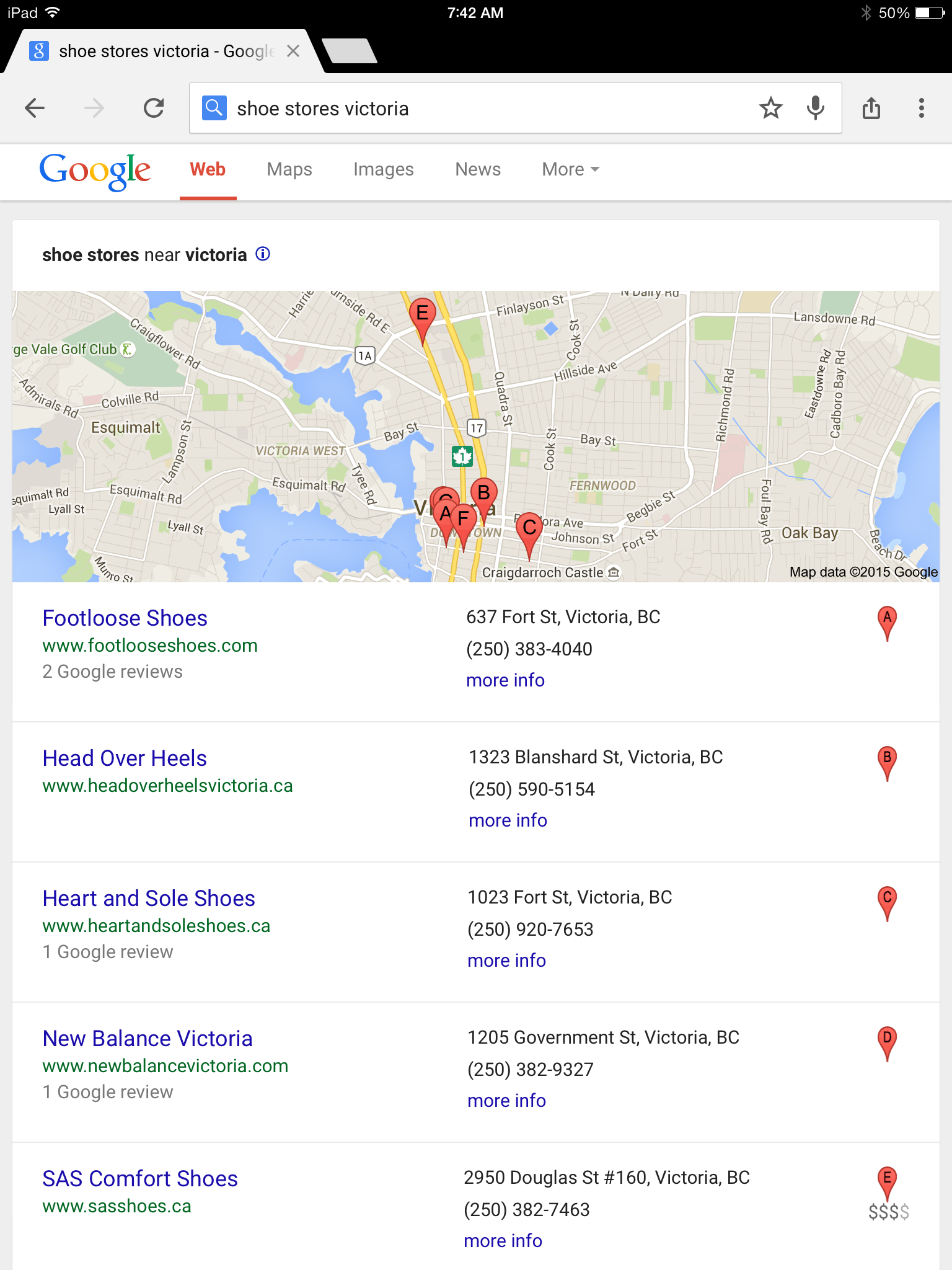The image depicts an iPad screen displaying a map interface on Google Maps at 7:42 A.M., with the device showing a 50% battery level. The map is centered around Victoria, British Columbia, and the interface includes Wi-Fi connectivity. Various navigational elements are visible, such as a left arrow, right arrow, and a refresh button. 

The top of the screen features red annotated text "E", and the bottom displays similar annotations "A", "F", "B", "C". On the map, you can see different shades of gray, green, and black indicating various terrains and streets, with prominent labeling in white text.

Points of interest are marked, including Frederick Castle and businesses like Footless Shoes located at 637 4th Street, Victoria, B.C. (www.footlessshoes.com, phone number 250-383-4040), Headoverheels at 1323 Blanchard Street, Victoria, B.C. (www.headoverheelsvictoria.ca, phone number 250-590-5154), Heart and Soul Shoes, New Balance Victoria, and S.A.S. Comfort Shoes. 

The map data is credited to Google, with the copyright dated 2015. Various Google services are accessible from the screen, including Web, Maps, Images, News, and more, with Web being highlighted in red. The interface prompts the user to choose directions towards Victoria, featuring icons such as a microphone and a half-star rating system.